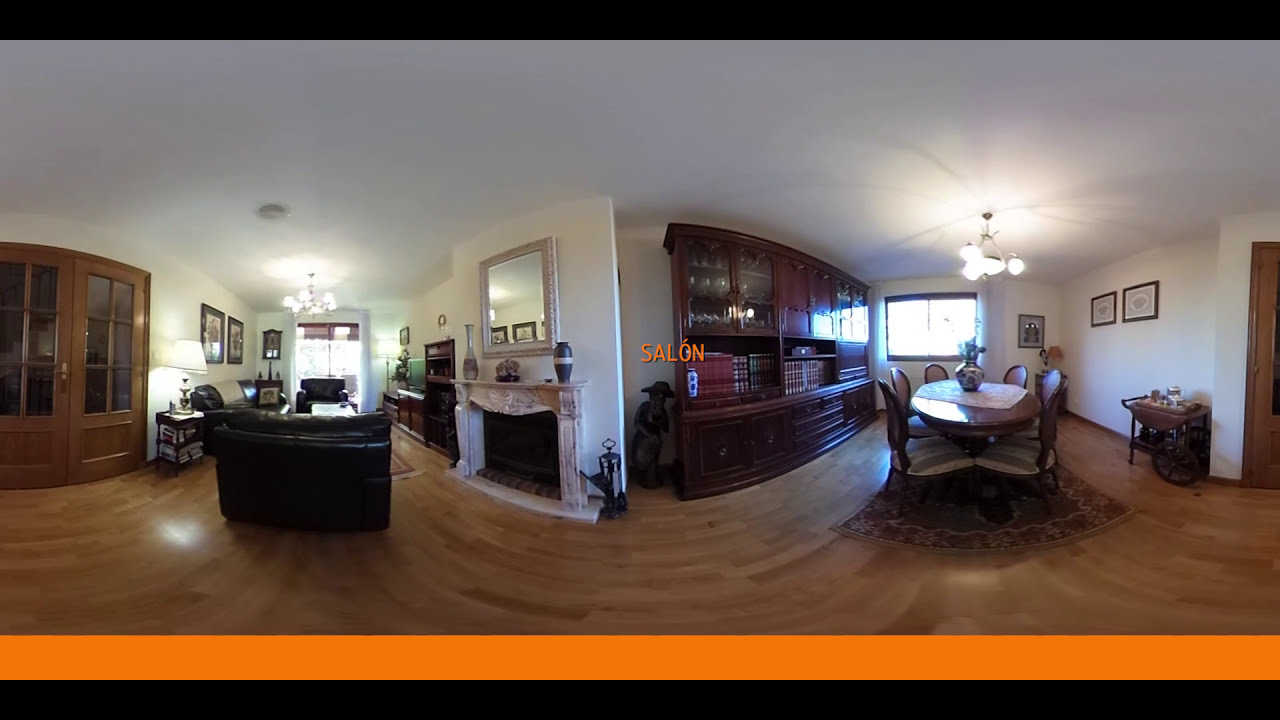The panoramic photograph showcases the interior of a bright, clean home, seamlessly blending the living room on the left and the dining room on the right. The living room, adorned with white walls and a light brown wooden floor, features a black leather loveseat and chair, a side table with a lit lamp, and two brown French doors on the left side of the wall. Above the fireplace, which is located on the right wall, hangs a large mirror, with vases adorning the mantle. Additional details include a coffee table and framed pictures enhancing the décor.

Transitioning to the dining room, which also sports white walls and light brown wooden flooring, we see an oval table set with six chairs situated on a rug, illuminated by a chandelier light fixture above. The dining area includes a window allowing ample natural light and a long curio cabinet filled with dishes and books. A small, black statue of a person with a hat, two framed pictures, and a cart with glasses on wheels further embellish the space. The image captures an overall sense of tidiness and brightness, underscored by the natural light streaming through multiple windows. A visible sign with the word “SALÓN” printed in orange accents the central area of the photo.